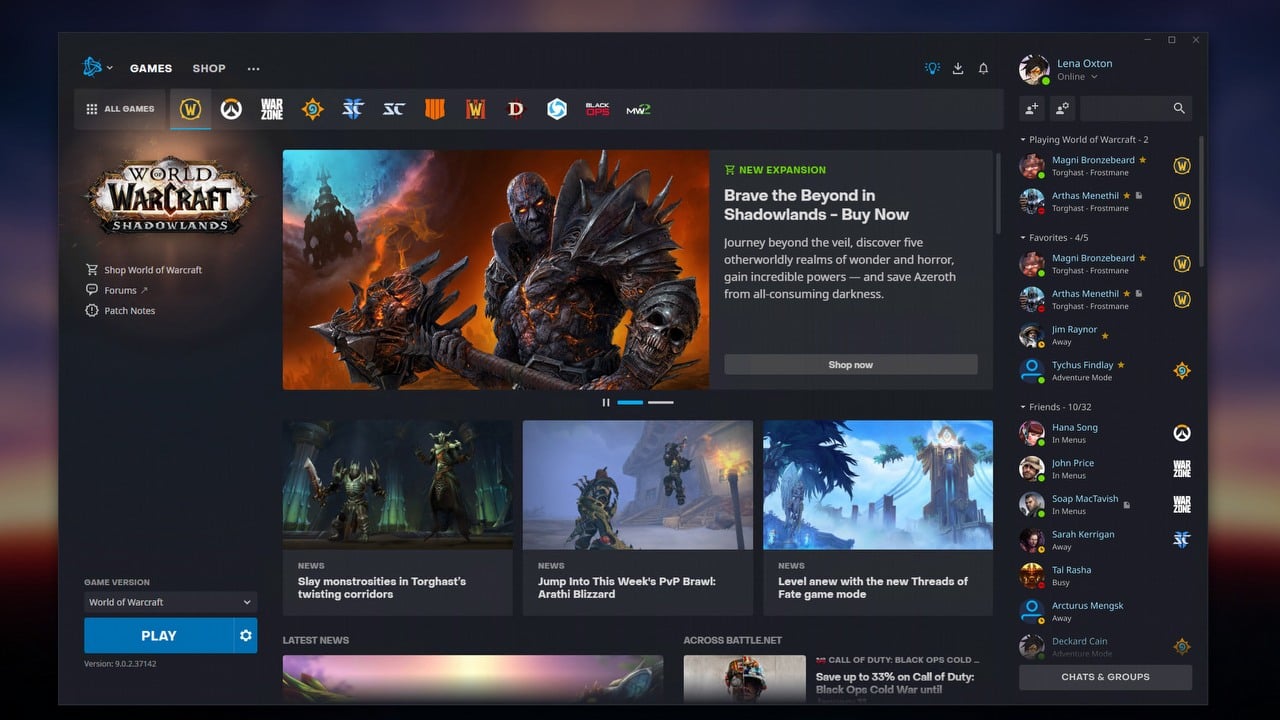This image showcases a detailed online gaming interface, presumably for "World of Warcraft." On the far left, a website menu is visible, with the blue "World of Warcraft" icon prominently displayed in the top-left corner. Beneath this, there are menu options labeled "Games" and "Shop." The background is dark gray, contrasting with the even darker gray of the main image.

Directly below the "World of Warcraft" title are three options, rendered in very small white text. The central part of the image features a striking graphic with predominantly orange and brown hues, transitioning to blue at the top left. The character depicted is clad in black armor adorned with numerous spikes, especially around the shoulders, has a black face marked by piercing orange eyes, and wields a large, spiked mallet.

To the right of this character, the text reads "Brave the Beyond" and "Shadowlands," followed by a "Buy Now" button and a "Shop Now" option below it. Further down, there are three gaming articles. The right-hand side of the image displays a user profile picture, alongside a list of online friends that populates the entire right column.

At the bottom left of the interface, a blue rectangular "Play" button with white text is present. This detailed image effectively captures the comprehensive and immersive nature of the gaming platform's user interface.